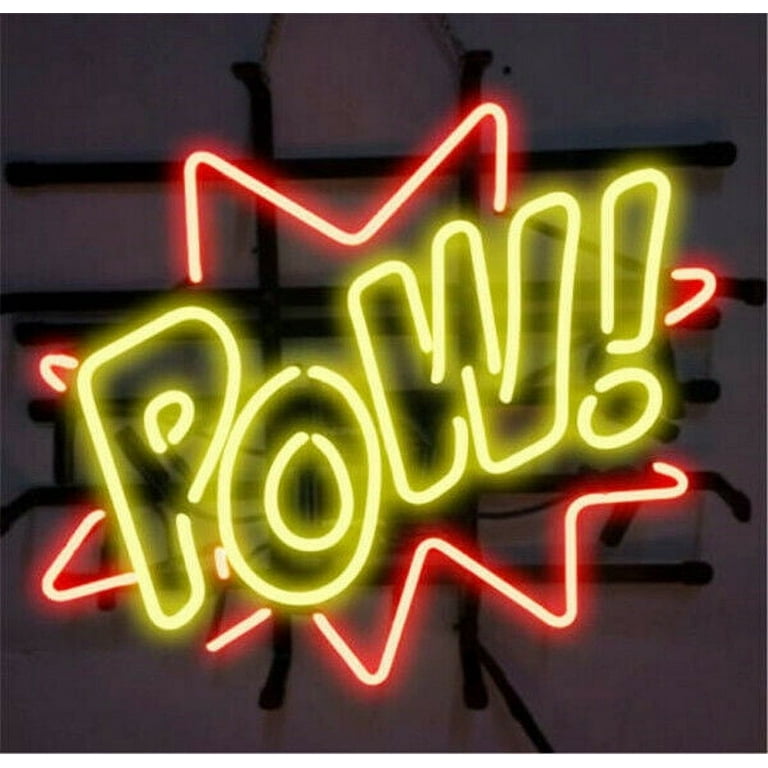The image showcases a square-shaped neon sign prominently featuring the word "POW!" in vibrant yellow neon letters, complete with an exclamation mark. Surrounding this central text is an explosion-like shape, lit up with dynamic, star-pointed red neon borders that give a sense of impact. The background is relatively dark and blurry, providing little detail beyond the sign itself, but hints at a grayish surface with black metal pieces, possibly a frame or structural support, crisscrossing behind. The vibrant neon elements make the sign stand out starkly against its subdued surroundings.